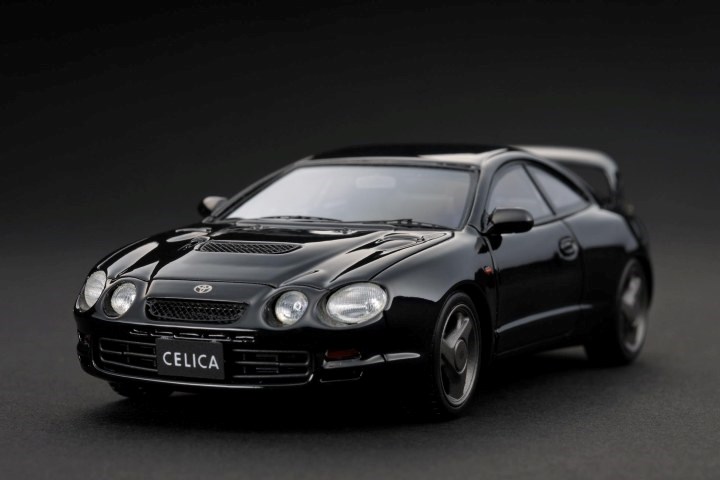This photograph showcases a sleek, black Toyota Celica sports car, prominently positioned against a black background that subtly blends with the charcoal gray ground beneath it. The vehicle, stationary and angled at approximately 45 degrees, faces slightly towards the lower left corner of the image, with its left front headlight and tire closest to the viewer, while the rear right tire remains hidden from view. The car's body is remarkably shiny, reflecting light off its surface.

The Celica features a distinctive rear spoiler and a sharply angled windshield, sloping back at about 50-60 degrees. Its front end sports four headlights: two oval-shaped outer lights and two slightly smaller, circular inner lights, all of which are off. The iconic Toyota logo, circular with intricate design elements, is positioned prominently between the headlights, just above the front fender. A license plate at the front of the car reads "CELICA" in bold, white, all-capital letters.

Other visible elements include a single driver's side door, silver hubcaps with triangular patterns, and sporty wheel rims with a center and three pillars angling towards the wheel. The overall composition, devoid of surrounding context or human presence, accentuates the car's glossy, aerodynamic form and advanced design features.